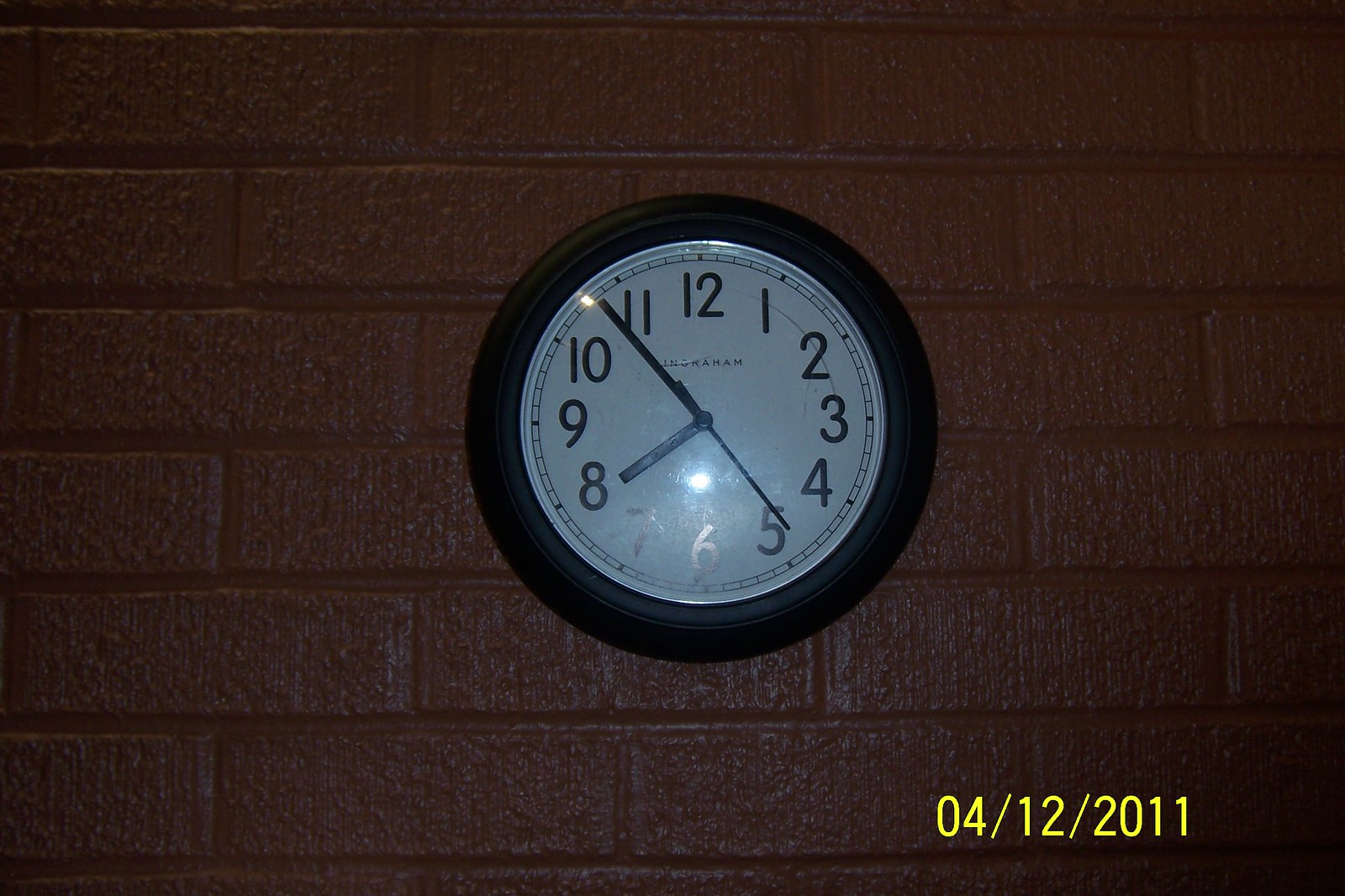The image features a circular clock mounted on a brown brick wall. The wall itself appears to be constructed from bricks that have been painted brown. In the bottom right corner of the image, the date "04-12-2011" is displayed in yellow. The clock has a plain white face with black numbers from 1 to 12 around its circumference. The time shown is approximately 7:54, with the hour hand, minute hand, and second hand all colored black. The clock's frame is a simple, black circular disk with a modest, slightly routered design, adding a touch of subtle detail to its otherwise straightforward appearance.